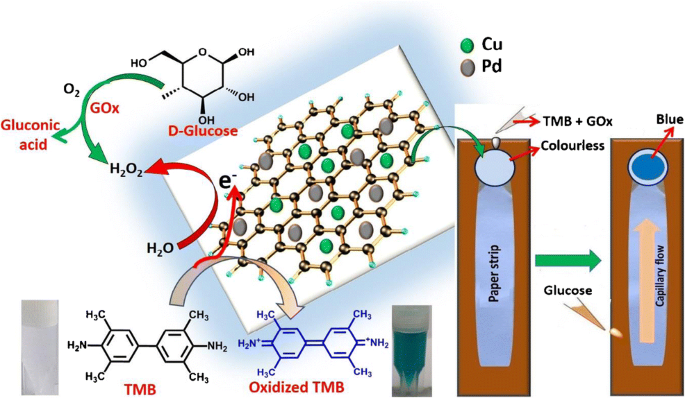The image illustrates a complex chemical process, likely depicted in a scientific poster, showing the breakdown and interaction of molecules. Central to the image is a horizontal white rectangle angled in the middle, displaying three-dimensional representations of molecules. These representations feature golden lines connecting golden balls, forming structures that include hexagons with green and gray balls atop. This central image is surrounded by curved red arrows labeled "H2O" and "gluconic acid," and green arrows with labels "GOX" and "D-glucose." Additionally, black hexagons marked "OH," "HO," and "O" detail further molecular elements.

In the upper right, a green circle mirrors the central molecules, labeled "Cu" for copper, and below it a gray circle labeled "Pd" for palladium. To the right, two vertical orange rectangles with blue cutouts are aligned, each designated as part of a testing process; the left one labeled "paper strip" and the right as "capillary flow," with green arrows connecting them and indicating the presence of glucose. At the bottom left, red text identifies "TMB" and "oxidized TMB," signifying changes observed in the molecular structures.

This detailed layout aims to illustrate the chemical interactions, particularly how various elements and compounds, such as glucose and copper, play a role in molecular transformations, possibly for a biochemical or diagnostic application.